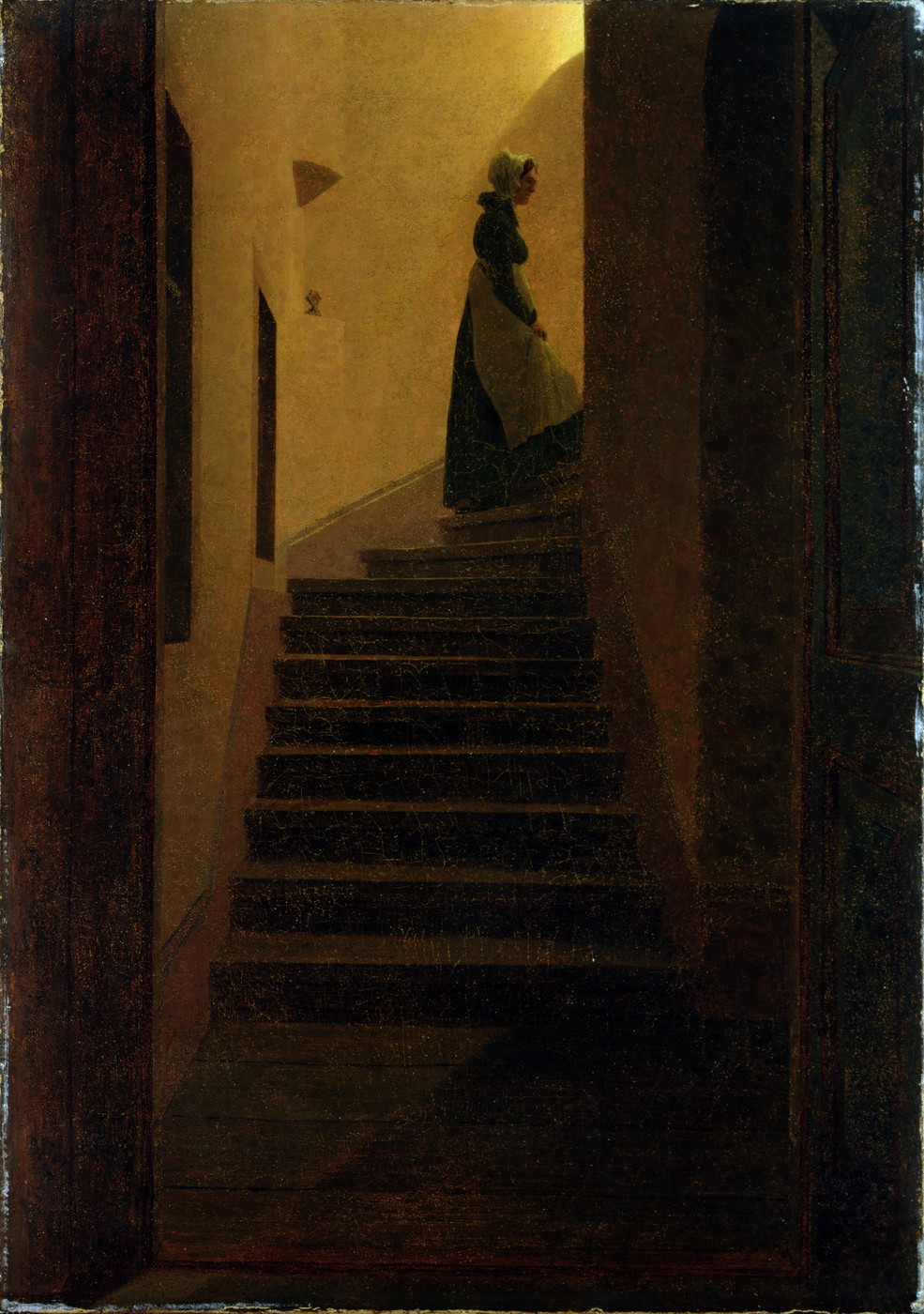This tall, rectangular painting, reminiscent of the style of Rembrandt and the Dutch masters of the 15th and 16th centuries, is a masterful depiction of a woman ascending a dimly lit staircase. The dark brown wooden walls on either side form an entryway to the staircase, which begins at the bottom of the image and ascends towards the center before turning behind a grayish orange wall. These walls are a lighter, muted yellow, adding to the painting's overall subdued and shadowed ambiance. At the top of the staircase, as it turns to the right, stands a woman dressed as a maid, viewed in profile. She wears a long, dark gown with long sleeves, a large white apron extending nearly to her feet, and a white bonnet on her head. With her hands clasped in front of her, she appears to be pausing momentarily before she moves out of the frame into the darker recesses of the stairway. The stairway is subtly illuminated with a golden hue, drawing attention to the figure of the woman and highlighting the detailed textures and depth of the scene.